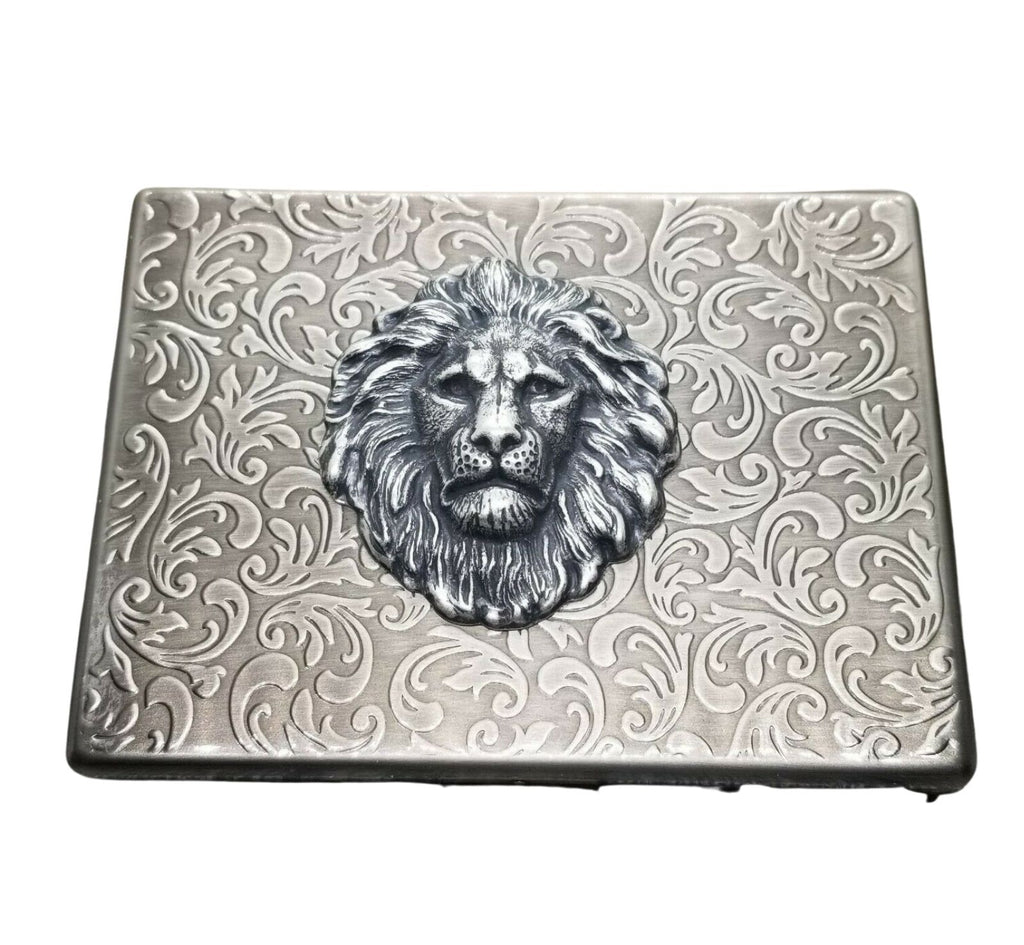This image showcases a stunning, antique silver metal piece with a brushed finish, almost square in shape. The surface is adorned with intricate, lighter silver filigree designs that resemble vines or floral patterns. The most striking feature is the large, three-dimensional lion head prominently positioned in the center of the piece. This detailed lion, crafted from the same silver material, has a realistic and somber expression, with a furrowed brow and closed mouth. Its eyes, especially the more visible left one, gaze directly at the viewer, and the eyes and mouth are particularly dark, almost black. The lion's mane is meticulously detailed, with a mix of black and silver hues that are darker than the lighter silver background. Below the lion’s nose, several dots represent where whiskers would grow, adding to the intricate detailing. The overall craftsmanship of the lion head, combined with the elaborate filigree, gives this historic-looking item a beautifully ornate and antique finish.